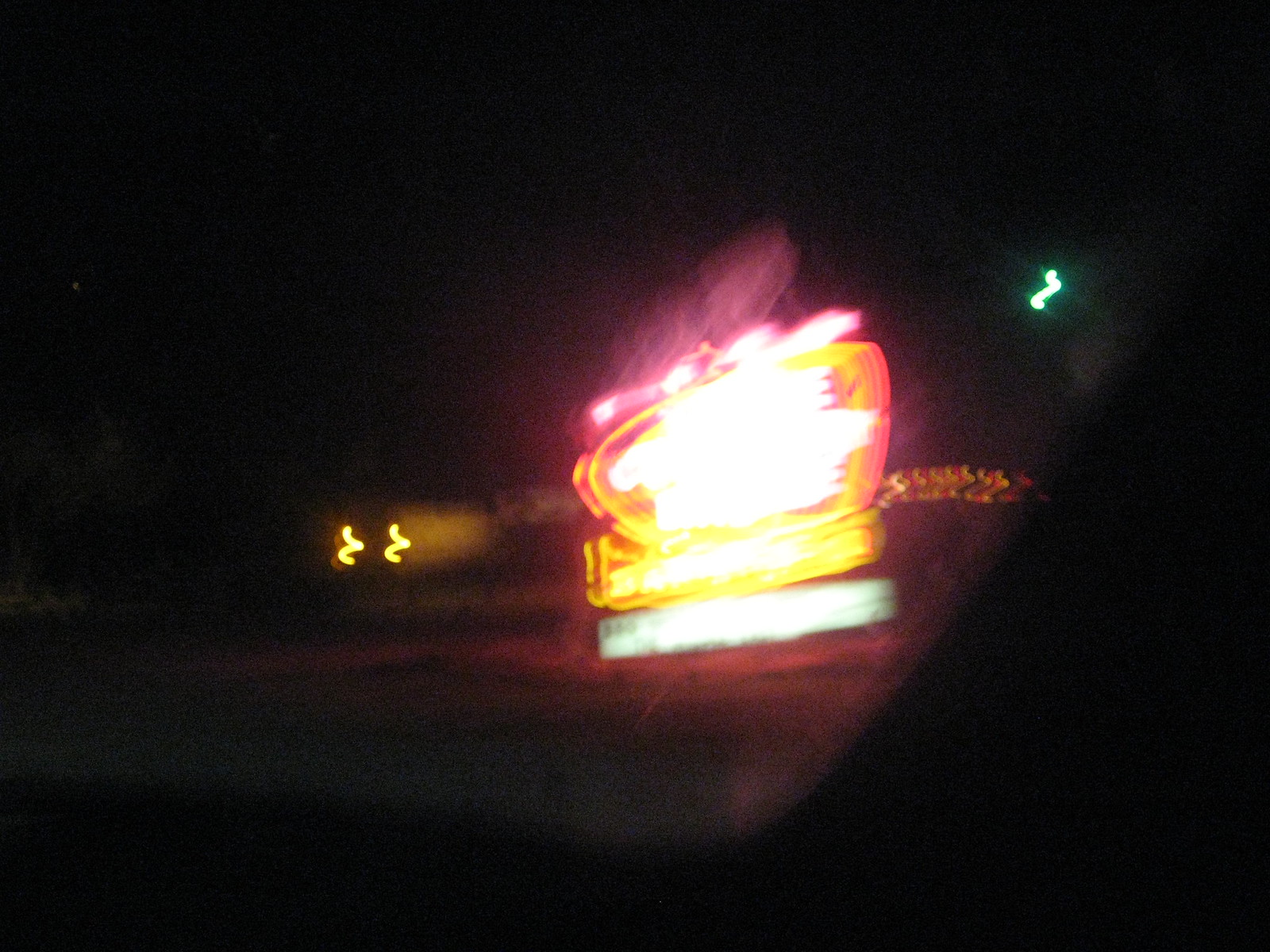The image is predominantly dark and blurry, with the majority of the frame enveloped in blackness. At the center, several bright lights pierce through the darkness. The uppermost light is a horizontal, pink strip that casts a pinkish reflection on the surrounding area. Below it, a circular or oval-shaped light displays a vibrant pink and yellow outline, with a bright yellow core. Further down, another horizontal strip of light is mostly yellow, accented by an orange outline. Directly below this, a greenish horizontal line appears, likely reflecting the lights above it. In the top right corner, a bright green squiggle is visible. Beneath this, additional lights form squiggly lines in yellow and red hues. Lastly, on the left side, two more yellow squiggles can be seen, adding to the chaotic yet colorful illumination in the image.